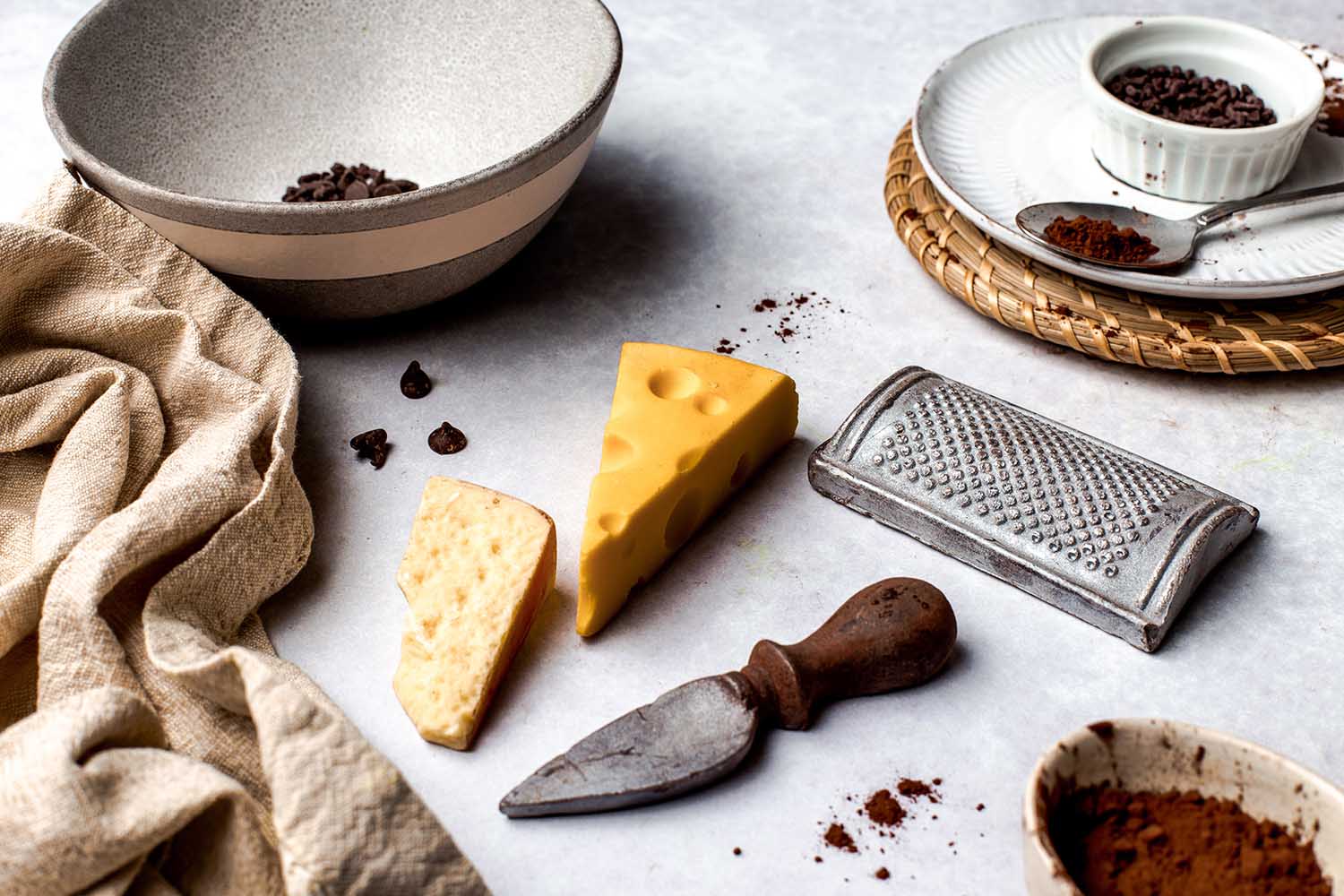This photograph showcases an elegantly arranged scene of cheese and coffee ingredients on a light marbled surface. In the foreground, two vibrant blocks of classic Swiss cheese, complete with iconic holes, rest centrally on the table. Accompanying the cheese is a rustic cheese knife with a wooden handle, and an older metal cheese grater lying adjacent. To the left, a textured brown cloth, resembling a towel or apron, hangs off the edge of the table, adding a cozy element. Just below the cloth, a stone or ceramic bowl, gray with a tan stripe, holds a small amount of chocolate chips, with a few scattered around it.

Towards the bottom right, a light brown or tan dish contains cocoa powder, some of which has spilled onto the table surface. In the upper right corner, a woven wicker trivet supports a white plate with an elegant gold trim. On this plate sits a small white saucer filled with finely ground coffee, some of which is also sprinkled around the plate and a small silver spoon laid nearby. This intricate tableau elegantly blends the rich textures and colors of cheese, chocolate, and coffee, evoking a sense of warmth and indulgence.